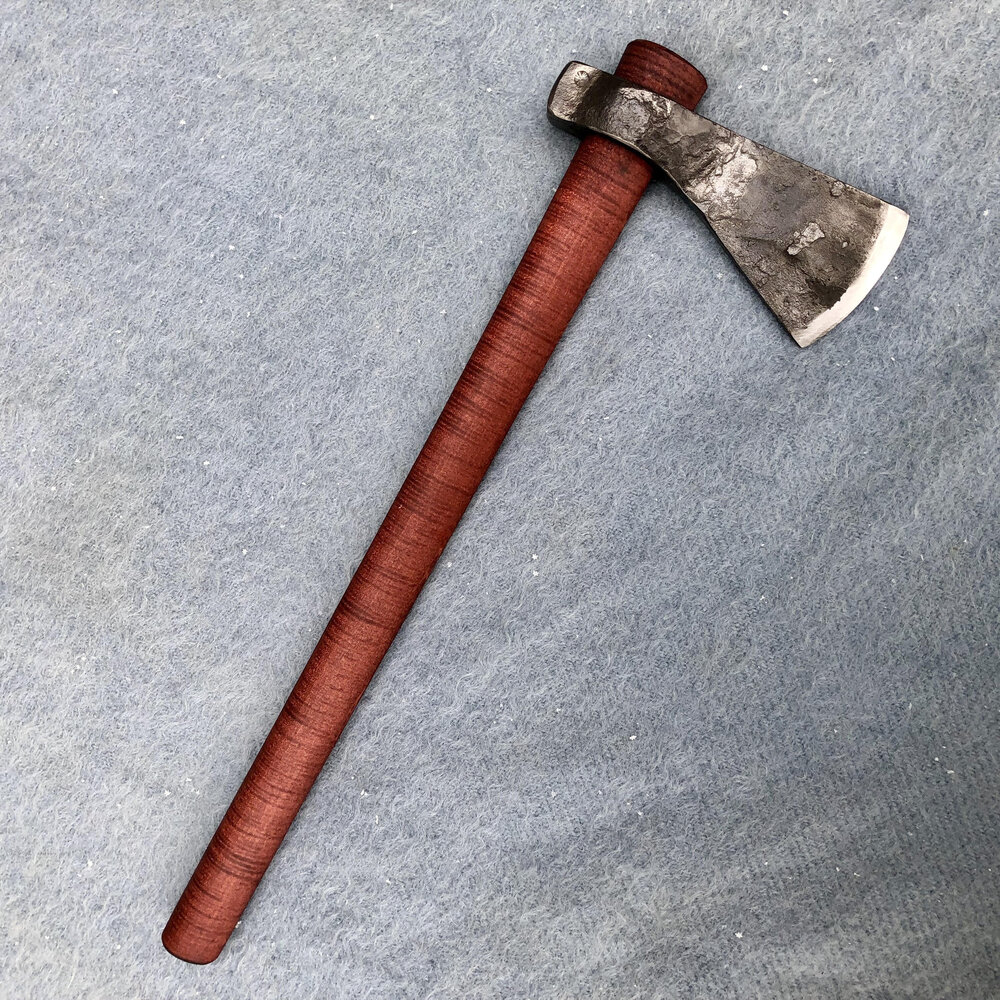This image features a detailed, close-up photograph of an axe laid horizontally on a light blue, felt-like fabric. The fabric displays distinct creases, particularly on the bottom right, top right, and center areas, with the left side appearing smoother. Specks of white dust are scattered from the lower right hand corner up to the axe's handle and around the top right where the axe is positioned.

The axe, seemingly medium-sized, comprises a wooden handle and a metal head. The handle, possibly made of cedar or redwood, is cylindrical, tapering to a smaller size at the bottom, and showcases distinct wood grains running horizontally along its warm, reddish-brown body, almost giving a spiral appearance. The top end of the handle, where the wood meets the metal, appears worn with splotches of white and gray.

The metal axe head is slightly angled downwards, predominantly gray in color with a rough patina, giving it an aged look. Despite this, the blade remains sharp and is illuminated by the light, shining almost silver at its edge. The axe head displays patches of dark gray, evidence of wear and usage, contributing to its weathered appearance.

Overall, this photograph captures the intricate details of a potentially ancient, well-used axe lying on a plush, light blue fabric surface.